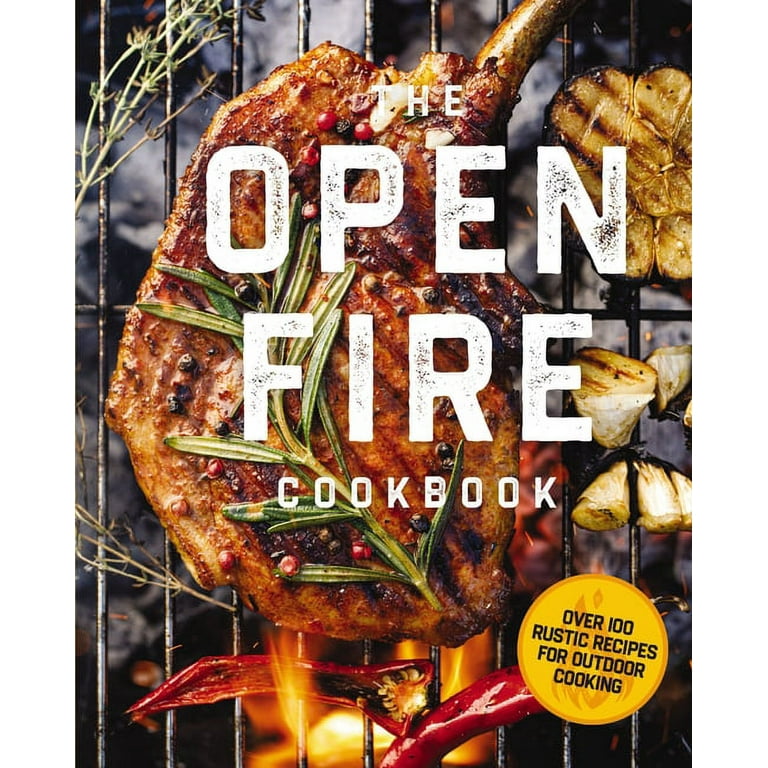This image depicts the cover of "The Open Fire Cookbook," prominently displaying the title in bold white font. The photograph on the cover spans the entire surface of the book and showcases a vibrant grilling scene. A grill rack laden with a variety of food items catches the eye, including a well-cooked steak, seasoned with barbecue sauce and resting on a bed of dill and red hot chili peppers. Surrounding the steak are roasted pieces of squash or zucchini, sprigs of thyme, rosemary, and cloves of garlic, adding to the rustic charm. At the upper right, a bone is visible, hinting at more grilled delights. A bright yellow circle at the bottom right of the cover highlights in black text, "Over 100 Rustic Recipes for Outdoor Cooking," inviting readers to explore the enticing world of open fire cooking detailed within the book.